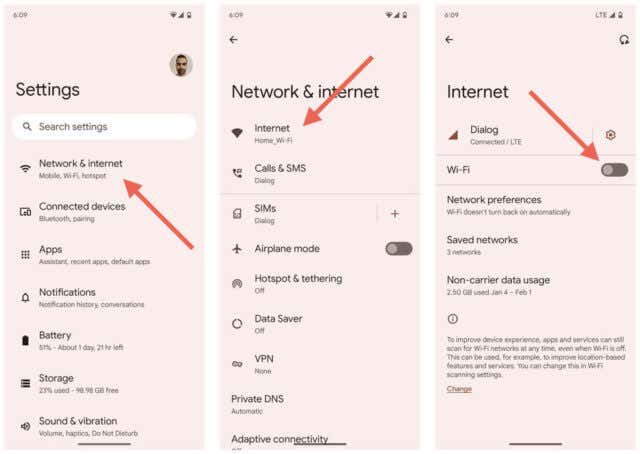This image set consists of three screenshots of a cell phone screen placed side by side, each with a consistent pink background. 

1. **First Screenshot:** Displays the "Settings" menu, highlighting the "Network and Internet" option. A red arrow directs attention to this option. Below it, other menu items like "Connected devices" and "Apps" are visible.

2. **Second Screenshot:** Shows the "Network and Internet" screen with a red arrow pointing at "Internet". The background remains the same pink shade as before.

3. **Third Screenshot:** Focuses on the "Internet" screen, pointing at the Wi-Fi toggle switch with a red arrow. Additional details in this screenshot include various network preferences, such as "Wi-Fi doesn't turn back on automatically", a list of saved networks (three in total), and data usage statistics ("2.5 GB" from January 4 to February 1).

Each of these images uses a light pink background and black font. The consistent use of red arrows serves to guide the user through the process of navigating from the main settings menu to enabling the Wi-Fi toggle, likely as an instructional guide on how to turn on Wi-Fi on the device.